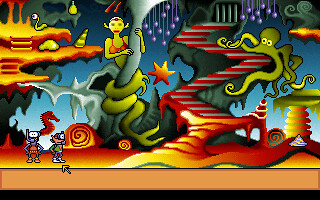The image appears to be a vibrant, colorful scene, possibly from a point-and-click video game or a highly stylized mural. Dominated by a pixelated yet intricate art style, it features a myriad of fantastical elements in an alien-like environment. At the center stands a green cartoonish imp-like character, whose long tail or protrusion is coiled around a beam or stalk. To their left, there is a platform resembling a red and yellow cliff. Further left, some red duck or dinosaur-like creatures are visible, along with a solitary yellow snail which adds to the whimsical ambiance.

On the right side of the image, a winding green branch with red steps leads upwards towards a blue sky, akin to a walkway. Perched on these steps is a green octopus with round legs. Nearby, a toadstool with a green top and yellow and green striped stem adds to the scene's otherworldly flora. Below all these elements, at the very bottom of the image, a beige, almost orangey line runs horizontally, accompanied by a slimmer black line, which might mark the edge of the mural or painting.

The scene also depicts two pixelated characters standing on this gradient of beige to orangey-tan terrain, with a yellow cursor at the lower right, hinting at an interactive video game interface. Above them, a snake-like creature with an eyeball for a head rests on a precipice, while a snake woman, wrapped around a column, emerges from the background, exhibiting an orange or reddish top. The overall backdrop transitions from light blue to dark blue, further enhancing the image's fantastical and surreal atmosphere.